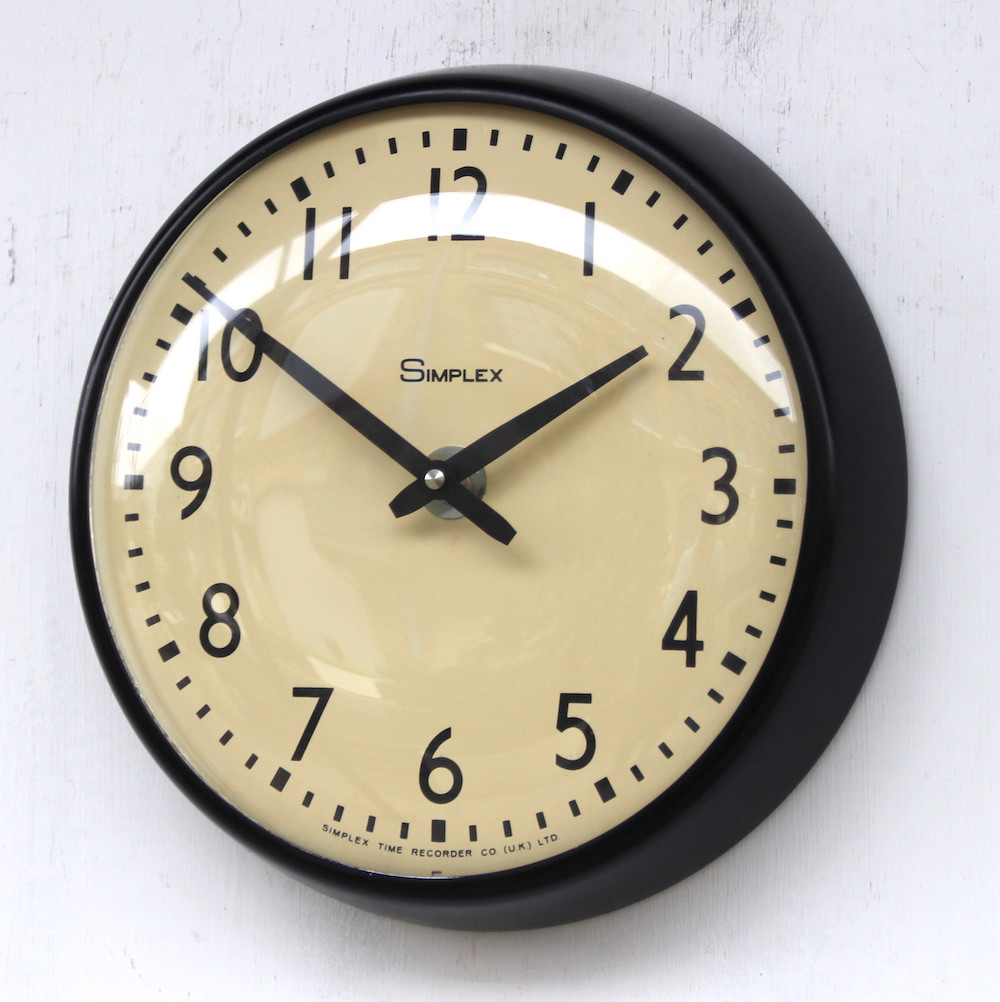A round clock with a black case is prominently mounted on a slightly scratched white plaster wall, which also bears faint pencil marks. The clock's worn appearance adds a touch of antiquity to the scene. Its beige face features clearly readable black numbers, complemented by matching black minute and hour hands. Positioned just above the clock hands, the brand name "Simplex" is displayed in black text. The clock's plastic cover is slightly convex, reflecting the overhead light source. At the very bottom of the clock face, beneath the numbers, the inscription "Simplex Time Recorder Company (UK) Ltd." can be discerned, further emphasizing the clock's vintage charm.